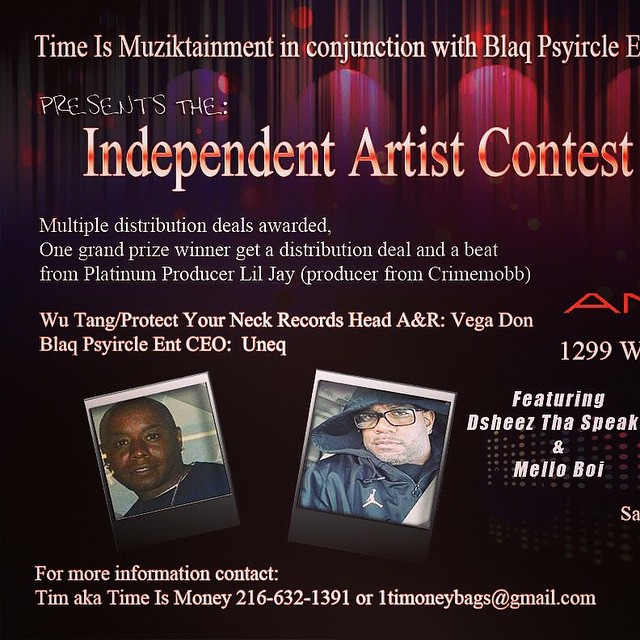This image features a flyer with a black and red gradient background that depicts a stage with red curtains illuminated by three white spotlights. At the top, in white text, it reads "Time is Muzik-Tainment in conjunction with Black Circle presents the Independent Artist Contest." Below, it announces multiple distribution deals, with a grand prize winner receiving a distribution deal and a beat from Platinum Producers Lil' J of Crime Mob, as well as recognition from Wu-Tang's Protect Your Neck Records head A&R Vega Dawn, and Black Circle Entertainment CEO Unique. Two Polaroid-style photos of two Black men are featured: the left shows a bald man in a black t-shirt, and the right depicts a man in a black zip-up jacket with an Air Jordan logo, wearing glasses. Additionally, it lists featured artists "The She's," "The Speak," and "Mellow Boy." For more information, it directs to contact Tim, aka Time is Money, at 216-632-1391 or onetimemoneybags@gmail.com.